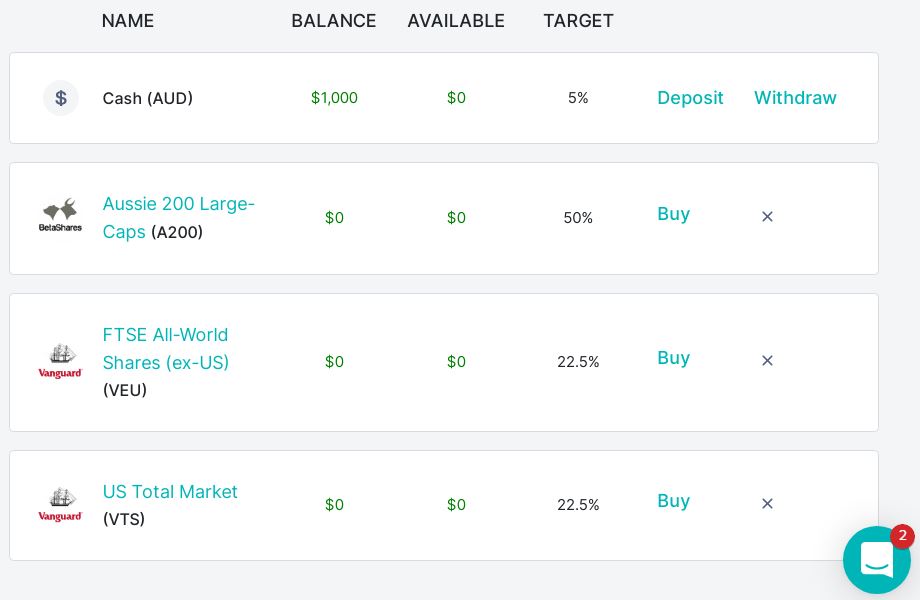This is a detailed screenshot of a trading application interface that displays information about various financial instruments, including cash, ETFs, and mutual funds. The interface is organized into several columns labeled "Name," "Balance," "Available," "Target," and options for actions like "Deposit" and "Withdraw."

At the top of the interface, there is a section for cash in Australian Dollars (AUD). It lists the Cash AUD category with the following details: 
- Balance: $1,000 
- Available: $0 
- Target: 5%
- Options: Light blue "Deposit" and "Withdraw" buttons on the right.

Below this section, there is a row featuring a logo of two animals—a bull and a bear—facing away from each other overlaying what appears to be the outline of a capital dome. The label next to this logo reads "Aussie 200 Large Caps (A200)," with details as follows:
- Balance: $0
- Available: $0
- Target: 50%
- Option: "Buy" (with no option for "Withdraw").

Further down, there is a red Vanguard logo featuring a clipper ship. The associated entry reads "Vanguard FTSE World Shares EXUS (VEU)" with these details:
- Balance: $0
- Available: $0
- Target: 22.5%
- Option: "Buy" (with no option for "Withdraw").

The subsequent entry has the same Vanguard logo but this time in blue. It details "Vanguard US Total Market (VTS)" with:
- Balance: $0
- Available: $0
- Target: 22.5%
- Option: "Buy" (again, with no option for "Withdraw").

In the bottom right-hand corner of the interface, within the last option row, there is a blue circle icon featuring a smiling speech bubble beneath it. This icon also has a red notification circle at its upper right corner with the number two inside it.

All elements in the interface are distinguished by thin pixel borders on a white background, presenting a clear and organized layout for users to manage their trades.